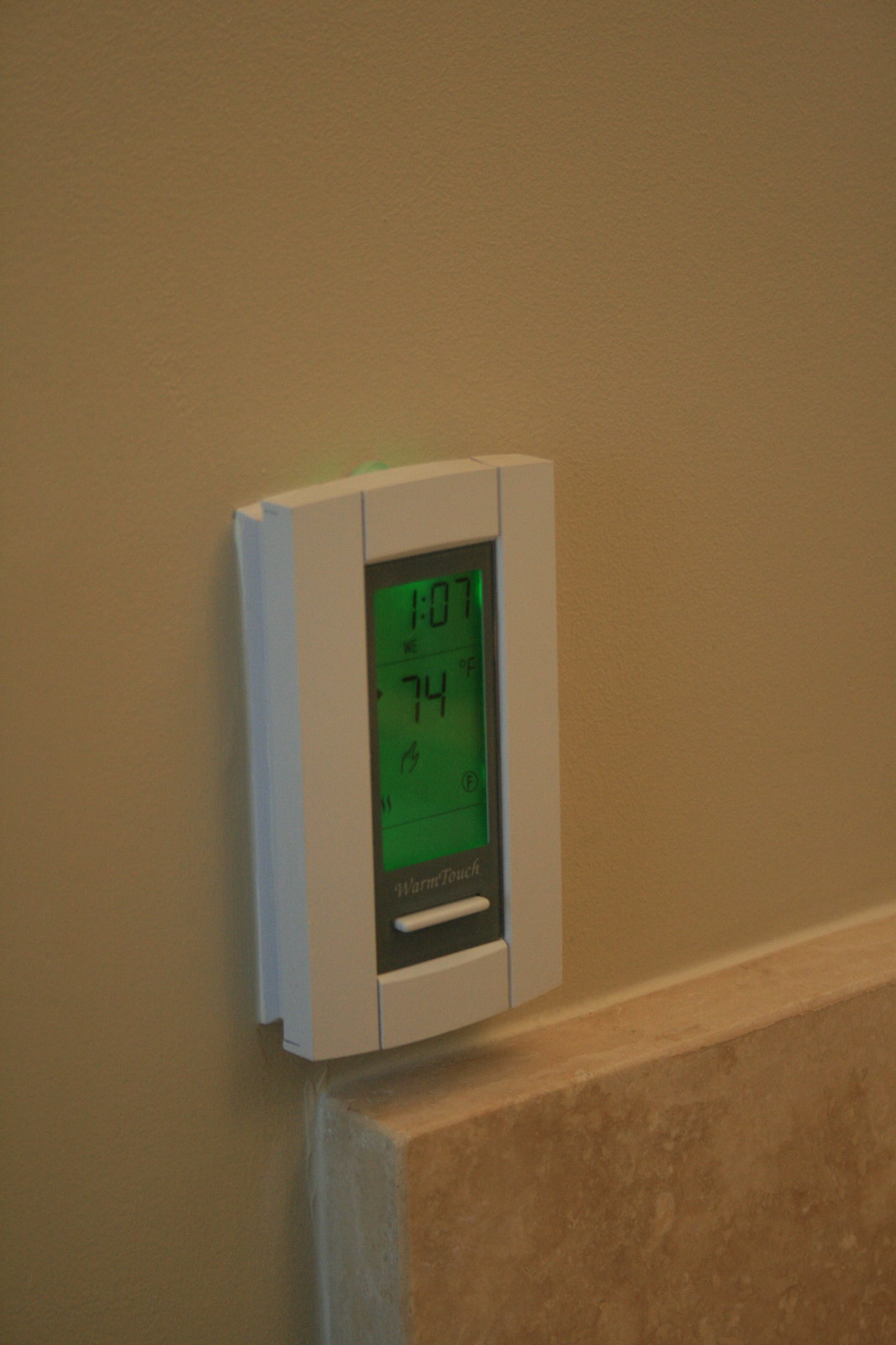This image depicts an indoor wall-mounted air conditioner controller. The wall is painted in a warm brownish hue. At the bottom of the image, a tile with a mix of brownish and whitish colors protrudes slightly. 

The air conditioner controller is small and rectangular, resembling the size and shape of a small mobile phone. The device is predominantly white, with a white border surrounding its edges. At the center of the controller, there is a screen framed by a grey outline. Below the screen, a long white button is positioned, with some text written above it in white lettering.

The central screen displays various data. A green light is illuminated prominently near the center. At the top of the screen, the number "107" is displayed, accompanied by an additional word below it. A black lining segments the screen, and the number "74" is prominently shown in the middle. Surrounding a hand gesture icon in the center are four smaller icons, each positioned on one of the four sides of the hand icon. 

The lower part of the screen remains plain, with no additional icons or text. Overall, the light on the controller is green at the center, and the numbers, along with other icons, appear in black.